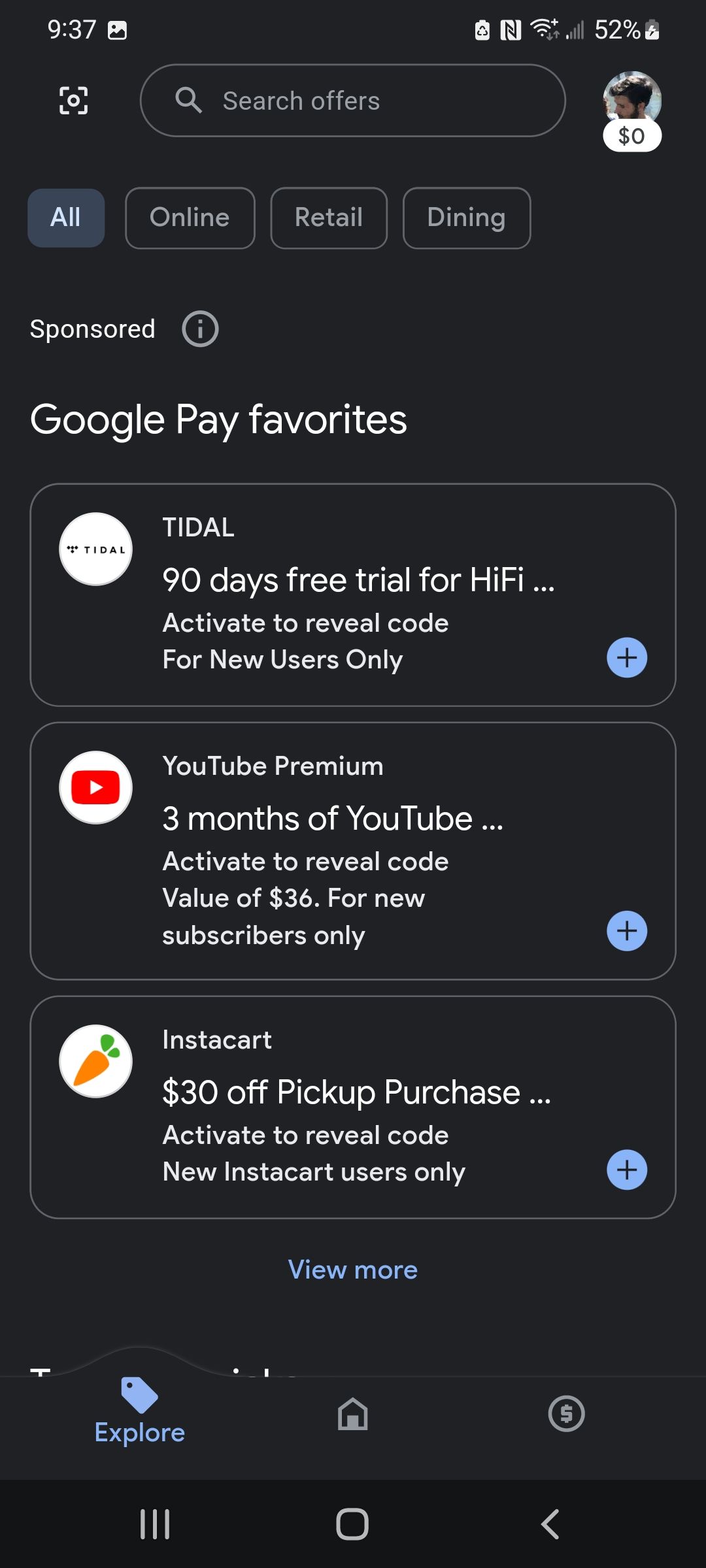In this intriguing UI display set against a solid black background, we see multiple elements arranged with precision. At the upper left corner, the number "937" is displayed in white text. At the upper right corner, a Wi-Fi icon and a battery indicator showing 52% charge signify active connections. Directly beneath the battery icon, there is a small, round photo of a young man in profile. He is adorned with a hat and sports a beard and mustache. Below his image, a speech bubble displays "$0."

Central to the layout, a search bar reads "Search offers" in gray text. Below the search bar are several category buttons labeled from left to right as "All," "Online," "Retail," and "Dining." The word "Sponsored" is prominently highlighted below these categories.

In large bold text beneath the sponsorship tag, "Google Pay Favorites" is labeled. The first featured option is a "90-Day Free Trial for Tidal Hi-Fi" with an "Activate to Reveal Code for New Users Only" prompt. Adjacent to this, the Tidal icon—a white circle with the word "Tidal" in dark text—stands out. In the lower right corner of this section, a small "+" button is situated. Underneath this, there's a promotional offer for "Three months of YouTube Premium."